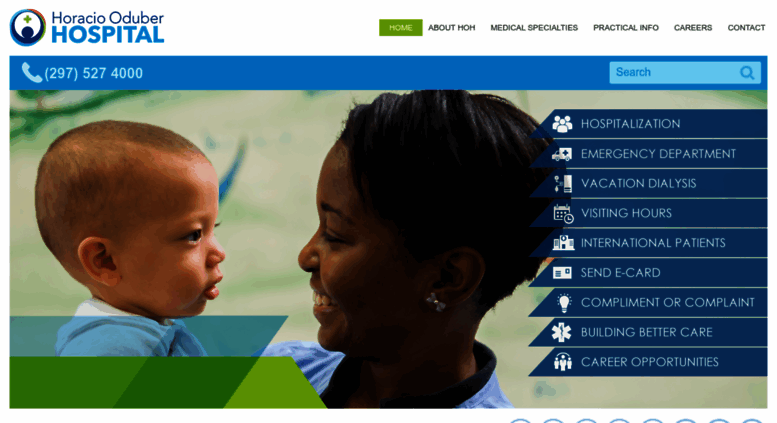This is a screenshot of the website for Horatio Ojibwe Hospital. The central image features an African-American woman with short hair, smiling warmly as she holds a young boy, approximately one to two years old, who appears to be of mixed race. At the top of the website, dropdown menus are visible, labeled as Home, About Us, Medical Specialties, Practical Information, Careers, and Contact. Directly below these menus, there is a blue rectangular section that contains a phone number and a search box. On the right side of the page, there is a comprehensive list of sections including Hospitalization, Emergency Department, Vacation Dialysis, Visiting Hours, International Patients, Send e-Card, Compliment or Complaint, Building Better Care, and Career Opportunities.